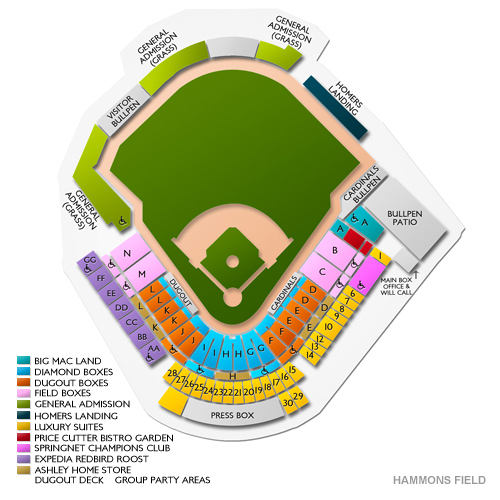The image portrays a detailed map of Hammond's Field, set against a white background. Central to the image is the stadium map, while the bottom-left corner features a color-coded table explaining the various sections of the stadium. 

The field itself is depicted in green, surrounded by a very light, almost pinkish outline. According to the table, different areas of the stadium are color-coded for easy identification:

- **Green areas**: Marked as General Admission
- **Pinkish areas**: Labeled as Field Boxes
- **Orange areas**: Indicated as Dugout Boxes
- **Blue areas**: Known as Diamond Boxes
- **Yellow areas**: Defined as the Luxury Suites
- **Golden areas**: Designated as Ashley Home Store Dugout Deck Group Party Areas
- **Purple areas**: Termed as Expedia Redbird Roost
- **Gray areas**: Including the Visitor Bullpen and Bullpen Patio

Additionally, there is a smaller box labeled Main Box Office and Will Call located near the larger map. The thorough detailing and color-coding effectively depict the layout and various seating options available at Hammond's Field.